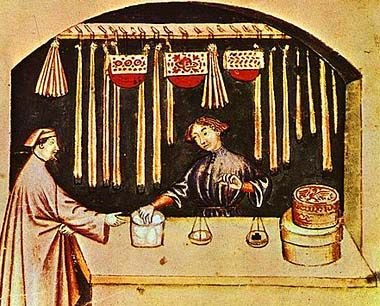The image is an artist's detailed depiction of a medieval marketplace scene, possibly an apothecary or a butcher's shop. At the center of the drawing, a merchant and a woman are engaged in a trade, standing by a wooden stall adorned with decorative ribbons. The merchant, dressed in a long reddish or pinkish robe and a distinctive cloth hat with a rim, reaches his hand toward the woman, who stands behind the counter. On the counter lies a scale with two items being weighed; one side holds a coal-like object, while the other possibly contains salt. Flanked by two tin containers, one of which is intricately decorated, the counter also features several beakers or Erlenmeyer flasks. Hanging behind the woman from a bar are identical pocket book-type containers and various other indistinguishable items, adding to the scene's rich, yet mysterious ambiance. The backdrop is dark, hinting at an interior space, but with no clear view of what lies beyond.